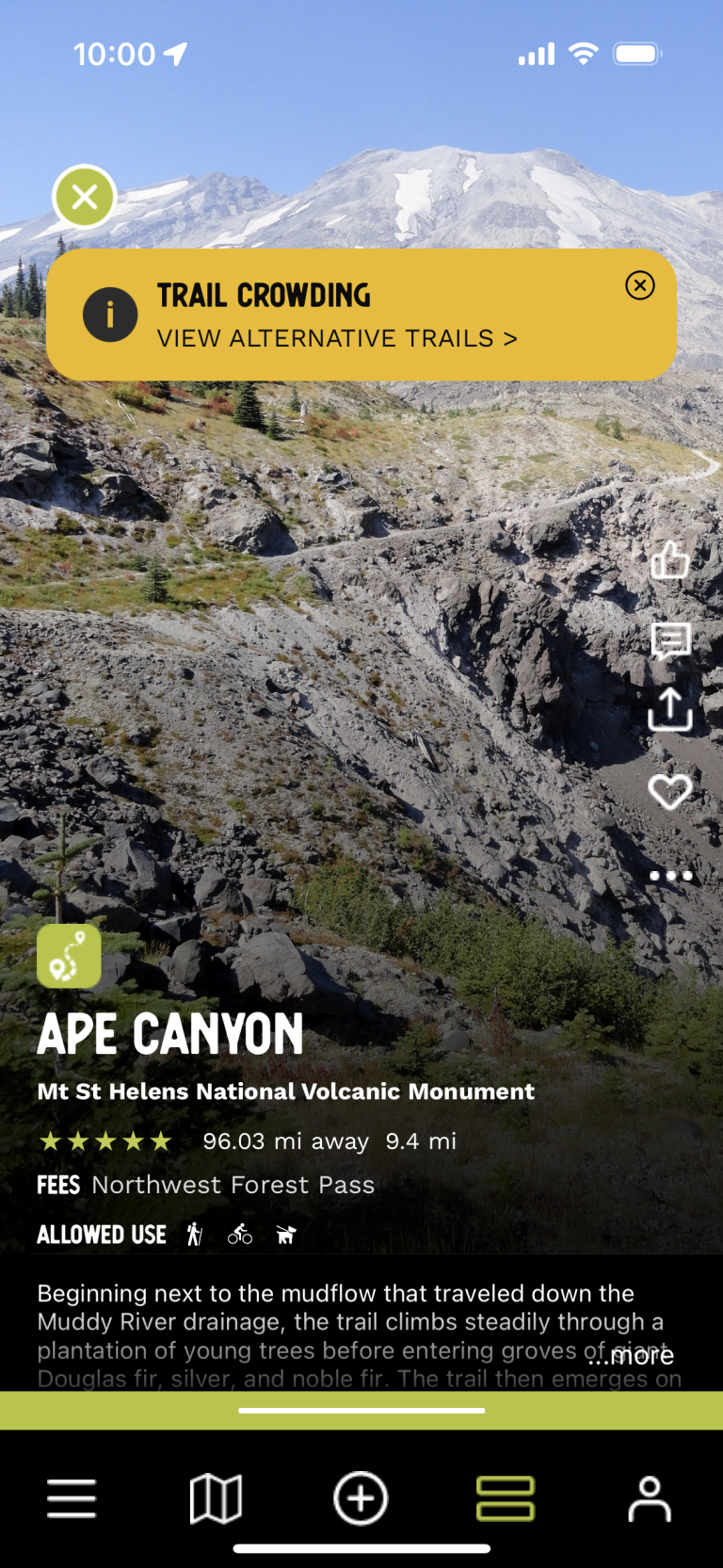Screenshot from a mobile device displaying a picturesque mountain landscape. The sky is a stunning shade of blue, providing a striking backdrop to the scene. Grey mountains topped with white snow dominate the middle of the image, descending into lush green grass and clusters of evergreen trees. At the top-left corner, the device status icons are visible: "10:00" with a GPS icon, followed by indicators showing full cellular service, Wi-Fi, and battery life towards the right.

In the upper section, a blue notification banner is present. Below, a yellowish rectangle with black text reads, "Trail Crowding View Alternative Trails," accompanied by a black circle with an "I" for information on its left. On the upper right corner, a black circle with an "X" is displayed for closing the notification.

Midway through the right side of the screen, a row of interaction icons is visible: a thumbs-up, comment, upload, heart/like, and an option symbolized by three dots. Centered on the screen in white text is the trail name "Ape Canyon," followed by "St. Helens National Volcanic Monument." Accompanying this, four gold stars, a distance of "96.03 miles," "9.4 M" for elevation, and a mention of "Fees, Northwest Forest Pass" give additional details about the trail.

A brief description follows, which is partially obscured but indicated by a yellow line with a white line in it and followed by three dots. Beneath this, icons for maps and other functionalities appear with two ambiguous symbols next to a profile image of a person on the right. All of these details are neatly framed against the scenic background, which enhances the informational display.